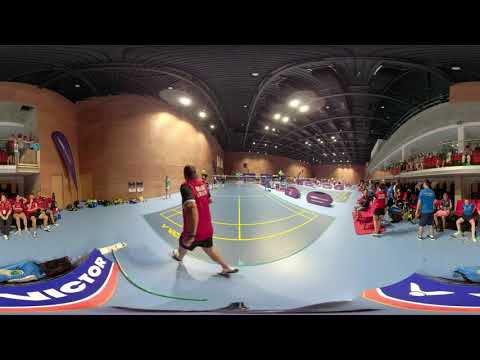The photo is an indoor color photograph of a sports arena, captured with a panoramic or 360-degree lens, resulting in a stretched and curved distortion. The arena features a dark gray court with yellow boundary lines, which appears suitable for either tennis or basketball, although the distortion makes it hard to distinguish. At the center, supported by two black poles, is a net with white and black sections.

The arena's structure is notable for its reddish brick walls and a dark gray ceiling adorned with multiple support beams and bright hanging light fixtures. The ceiling and floor are accentuated by black bars, indicating that this might be a still capture from a video. Additionally, there are distinct markings like the word "VICTOR" in white on a blue background and a V logo on one side.

On both the lower and upper levels, there are viewing areas filled with dark gray chairs, all occupied, indicating a well-attended event. In the middle of the distorted image, a male player dressed in a red vest over a black short-sleeve shirt and black shorts is visible, walking from right to left. The presence of similarly dressed individuals suggests this is a team event.